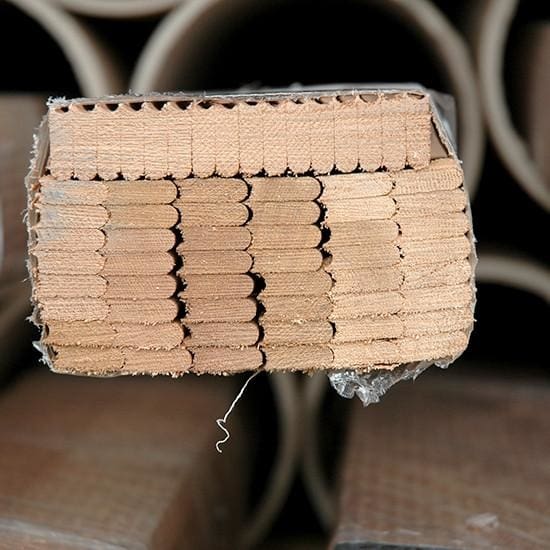The image shows a close-up of several stacks of small, beige wooden pieces that resemble old-fashioned popsicle sticks. The pieces are rounded on one side and feature notches on the other, suggesting they are designed to interlock, possibly for flooring or a similar purpose. These stacks, each boasting 48 interlocked pieces arranged in rows of 8, are tightly wrapped in transparent plastic, giving them an appearance of packaged goods. The photo is taken in portrait mode and hints at an industrial setting, likely a warehouse or factory, where the stacks are placed on a chair or amongst other items. The light wooden texture shows slight variations in shading, making it difficult to discern the exact material, though cardboard or some type of wood is plausible.